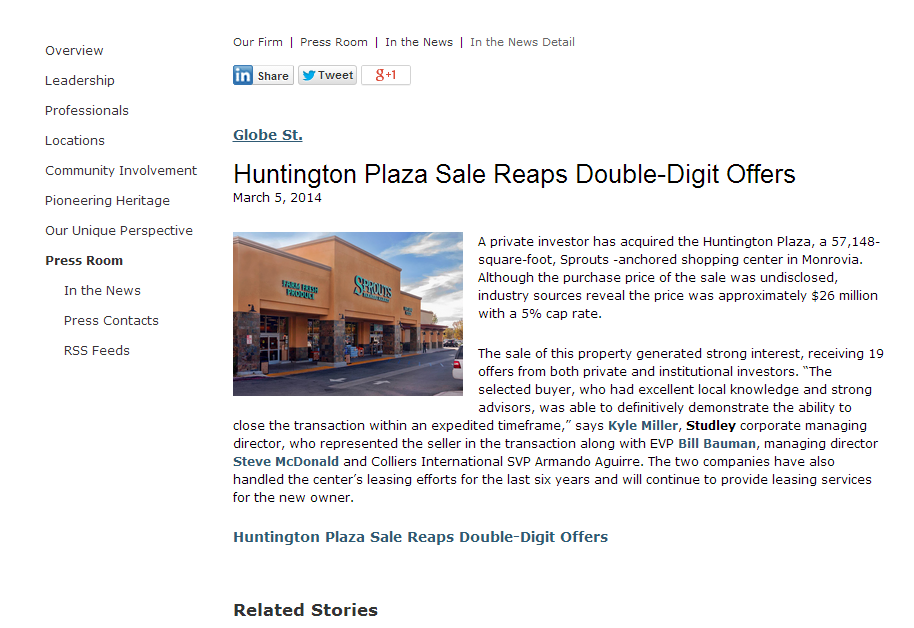A screenshot from an outdated news website is depicted. The upper section of the image showcases various navigation options and headings related to professional locations and communication, particularly focusing on heritage and unique perspectives. It also prominently features the "Press Room" in bold black text.

Towards the top-right corner, the image includes links to "Share on LinkedIn," "Tweet It," and "Google Plus," highlighting the dated nature of the content since Google Plus is no longer active. 

Central to the screenshot is an article from Globe Street with the headline, "Huntington Plaza Sale Reaps Double-Digit Offers," highlighted in bold black text. The article's date, March 5, 2014, is displayed in white text, confirming the period of the content.

The image portion includes a photograph of the Huntington Plaza, featuring a tan building decorated with white store names, set against a backdrop of a clear baby blue sky with scattered white clouds. 

Accompanying the image, the article notes that a private investor has acquired Huntington Plaza, a 57,148 square foot shopping center in Monrovia. While the details of the sale were not disclosed, it is approximated at $26 million with a 5% cap rate. The sale attracted significant interest from 19 potential buyers, indicating a robust market demand. Additionally, current leases are confirmed to continue for at least another six years.

The bottom left section of the image lists "Related Stories" in black text, providing readers with additional content options.